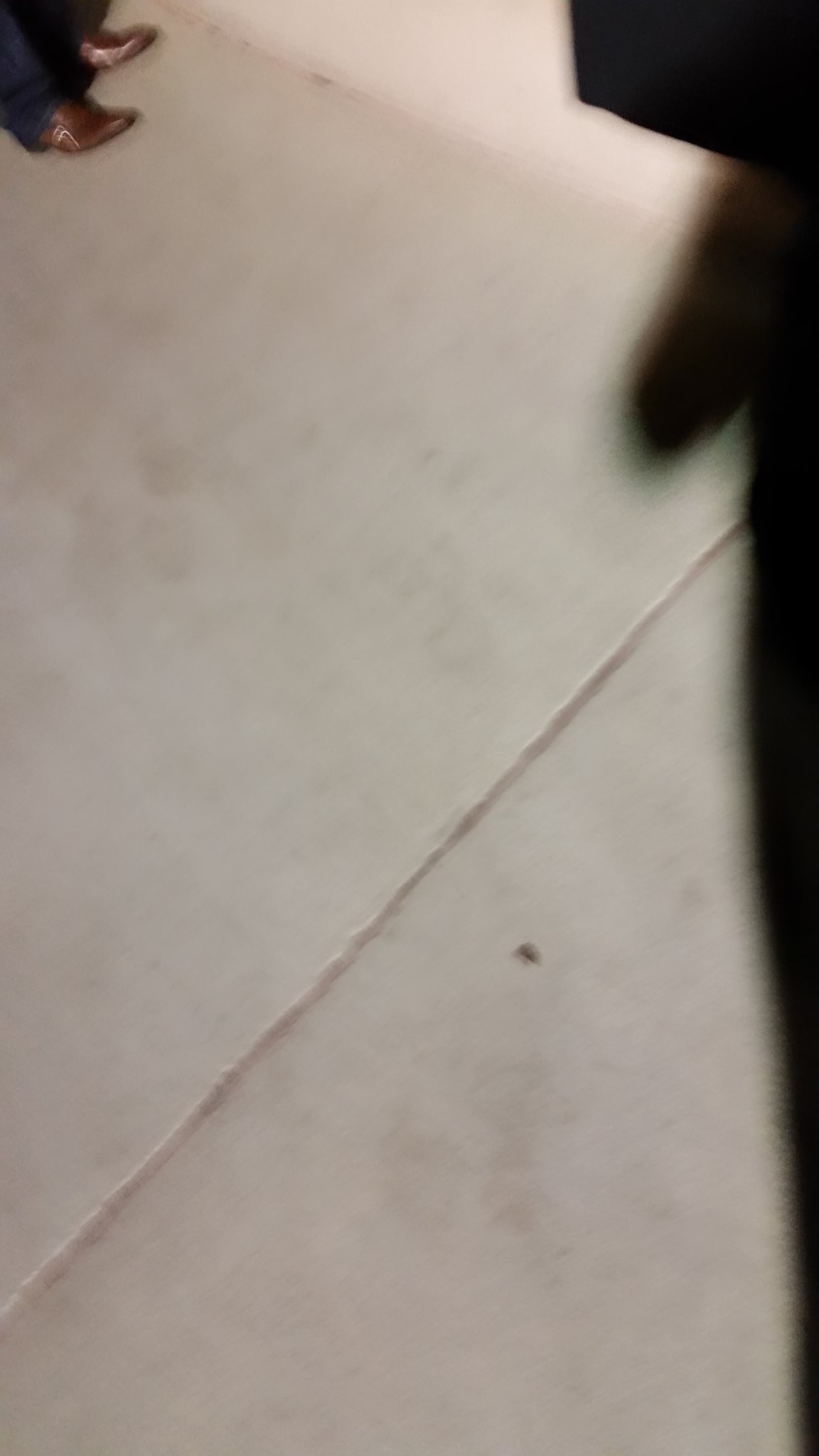This photograph appears to be an accidental shot of a concrete floor. In the top left corner, part of a person's attire is visible, revealing brown, pointy boots paired with either black or dark navy pants. The rest of the background features a concrete surface with a prominent divot line extending diagonally from the bottom left to the top right corner. On the left side of the image, there is a hint of another person, indicated by a dark, indistinct form. Additionally, a black rectangle can be seen at the top of the photo, along with a long, skinny line running vertically along the left edge.